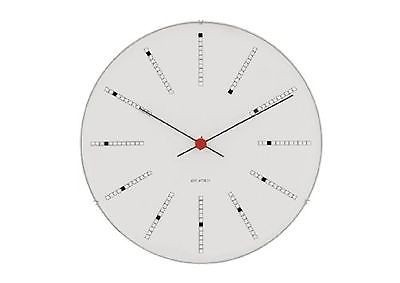The image depicts a clock face set against a white, solid background with a distinct, minimalist design. The circular clock face itself is entirely grey and bordered by a thin black line, giving it the appearance of being cut out or photoshopped from another source. Instead of traditional numbers, the clock features black rectangular dashes marking the hours, adding a modern and somewhat pixelated aesthetic. These dashes could be misinterpreted as tiny squares or even diamonds at first glance.

At the heart of the clock, where the hands pivot, there is a noticeable red dot. Two very thin black hands extend from this central point, with the longer hand (minute hand) pointing where the 2 would be on a traditional clock, and the shorter hand (hour hand) indicating where the 10 would be.

Additionally, there is some illegible text beneath the center of the clock, further enhancing the mysterious and stylized nature of the image. Overall, the absence of traditional numerals and the unique design elements suggest it may be an illustrated or digitally manipulated representation rather than a photograph of a real clock.